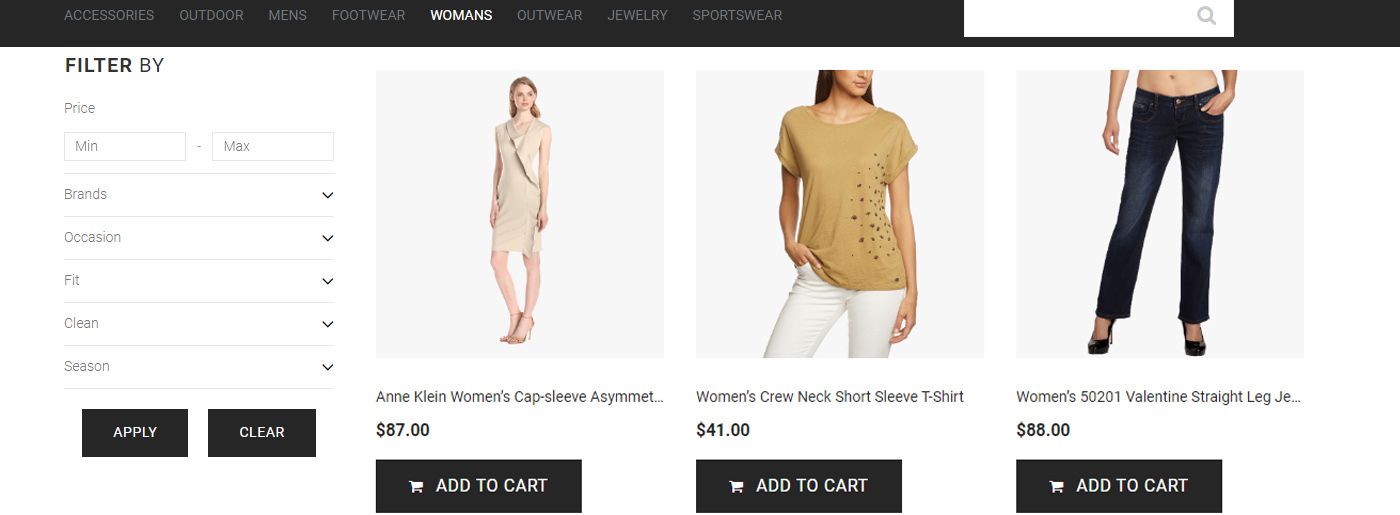The screenshot appears to be a mock-up of an e-commerce website. At the top, there is an unbranded gray navigation bar featuring menu options: Accessories, Outdoor, Men's, Footwear, Women's, Outdoor Jewelry, and Sportswear. The "Women's" category is highlighted. To the right of the menu, there is a search field.

Below the navigation bar, there is a filtering section with fields for price range (min and max), brands, occasion, fit, and season, accompanied by gray "Apply" and "Clear" buttons.

The main content area, set against a white background, displays three product options:

1. **First product:** A Caucasian woman with blonde hair, wearing a knee-length, cap-sleeve, asymmetrical dress. The product title reads "Incline Women's Cap Sleeve Asymmetrical..." but the description is cut off. It is priced at $87 with an "Add to Cart" button in gray.
   
2. **Second product:** A woman in a light brown top with patterned dots and white jeans. The product is described as a "Women's Crew Neck Short-Sleeve T-Shirt," priced at $41, and includes an "Add to Cart" button.

3. **Third product:** A woman wearing straight-leg jeans and high-heeled black shoes. The product title is "Women's 501 502-01 Valentine Straight Leg Jeans," priced at $88, with an option to "Add to Cart."

Overall, the website mock-up showcases a clean and minimalist design, possibly being developed as an e-commerce solution.